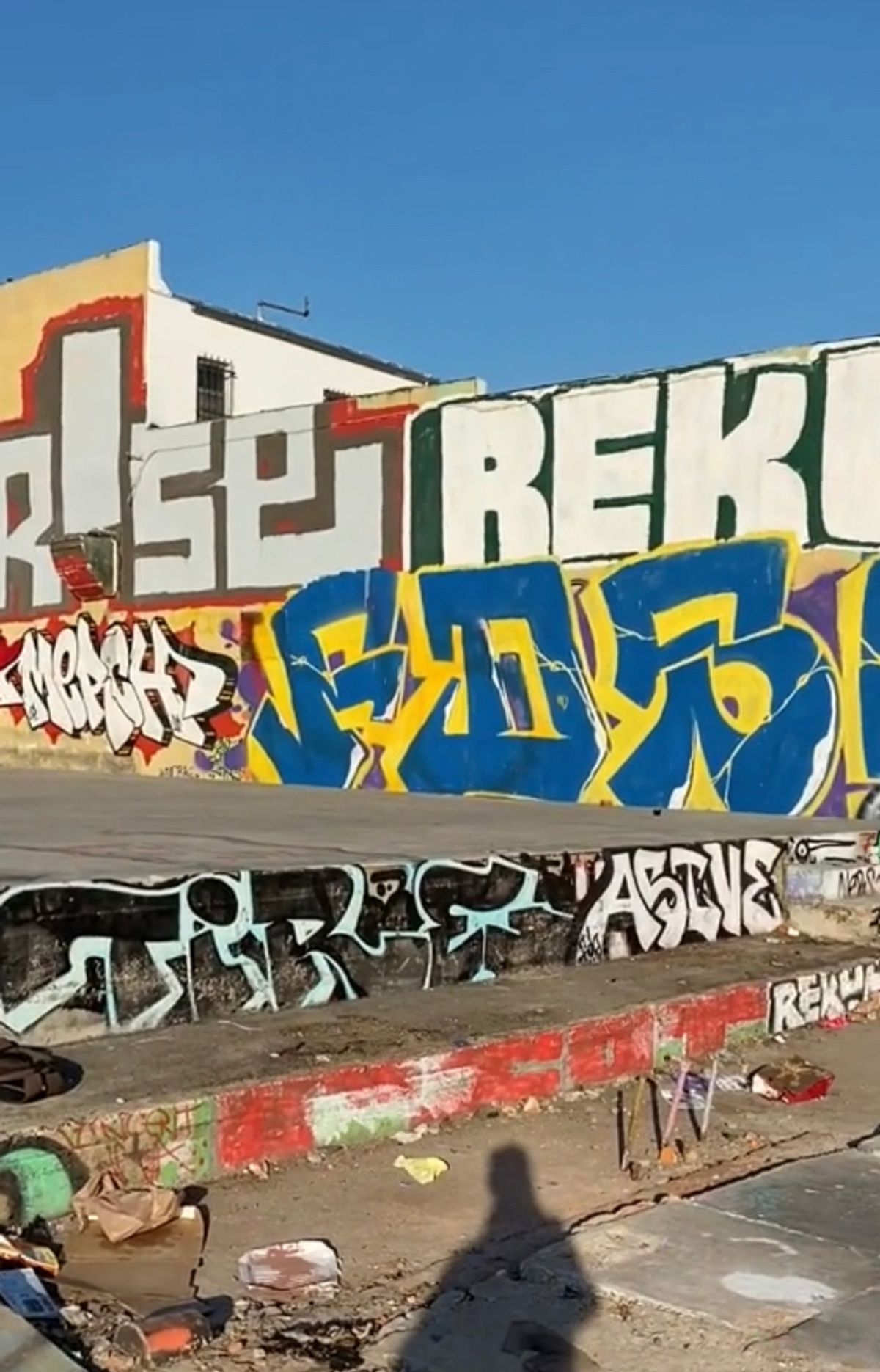The image captures a dilapidated, graffiti-covered building in broad daylight, set against a bright blue sky. The main structure is a two or three-story white building with a flat front facade, heavily adorned with layers of graffiti. Prominently, the upper part of the wall features bold, white graffiti letters spelling "R.E.K." The middle section includes a chaotic mix of blue and yellow designs with letters that are mostly unreadable, and some white and brown text that blend into the beige background, making them difficult to discern. At the foreground, a concrete slab sits about six feet high, leading to a set of crumbling steps, which are also adorned with graffiti. The area is littered with debris, including a plastic can and a brown paper bag, particularly noticeable on the lower left. Additionally, various metallic rods and stainless steel elements protrude around the area, adding to the disarray. The shadow of a person, presumably the photographer, is cast prominently in the center at the bottom of the image, adding a human element to the stark urban scene.